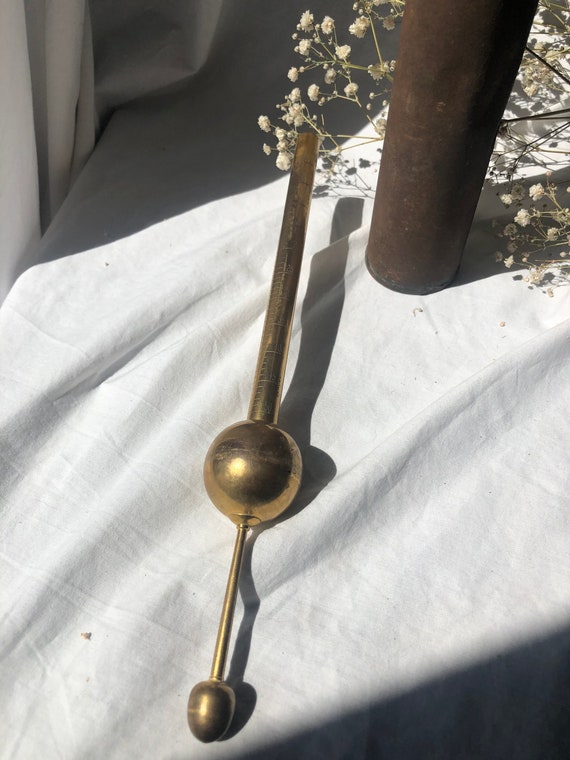The photograph captures a brass religious artifact, possibly used by a priest for ceremonial purposes such as baptisms or funerals. The artifact features a long rod, with a sizable round ball at the top, followed by a smaller rod, culminating in a raindrop-shaped tip. The elegant artifact lies on a slightly wrinkled white cloth. Adjacent to it is a bronze vase or urn, partially visible, filled with what appear to be cream-colored baby's breath flowers draping around it. The setting is indoors, illuminated by sunlight casting shadows through a window onto the light gray floor.